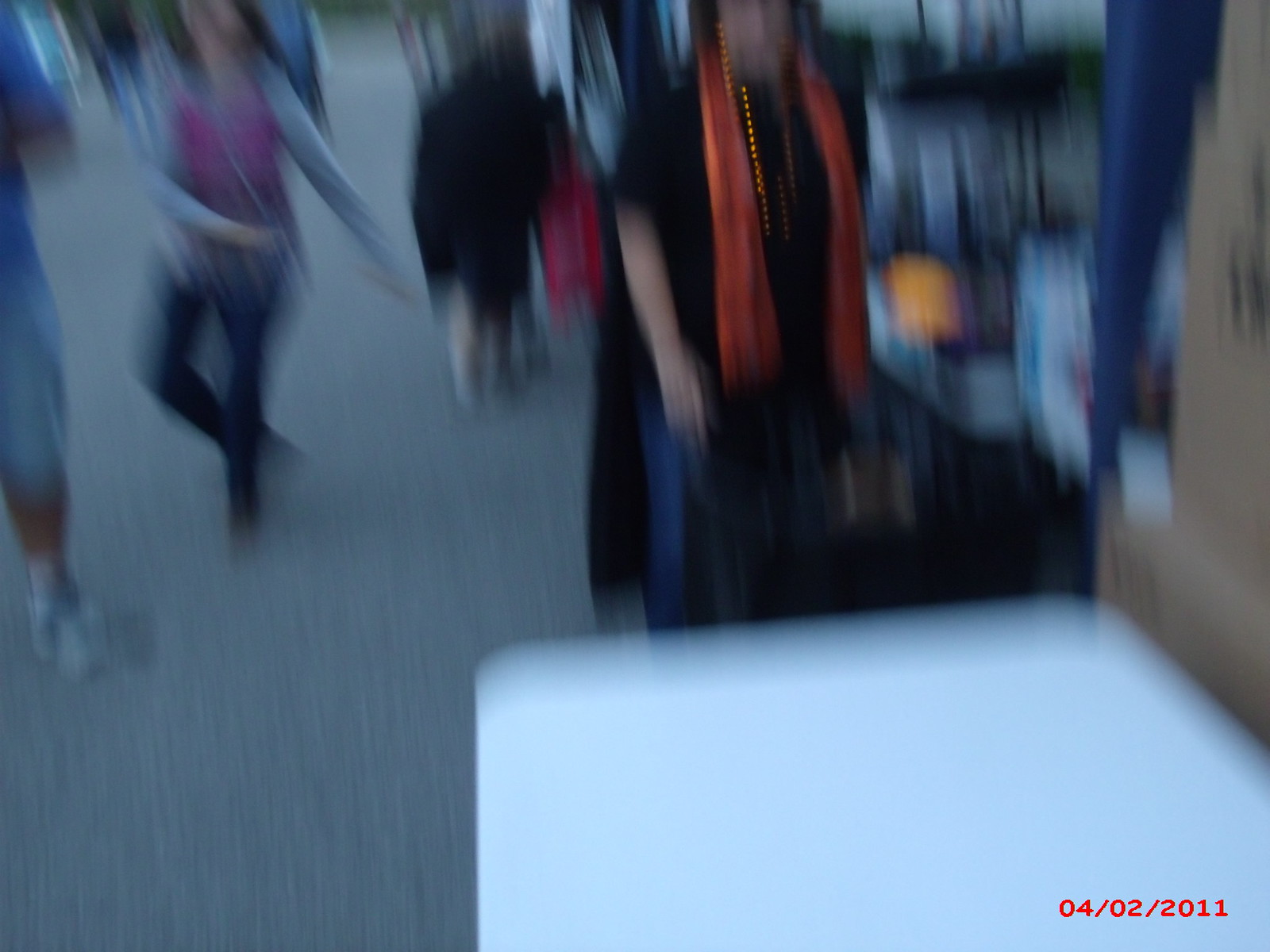This indoor, somewhat blurred photograph captures a scene predominantly viewed from an elevated angle. In the bottom right corner, a large white rectangular tabletop extends into the frame. At its end, the lower half of a woman's face and her body are visible; she is adorned in a short-sleeved black top paired with blue jeans and a reddish-orange scarf draped over her neck. She appears to be preparing to place a bag on the table. Adjacent to her on the right, a stack of brown boxes is discernible, suggesting a retail setting with hues of blues and whites in the background. 

In the upper left section of the image, another woman with long dark hair is caught mid-stride. She is dressed in a pink top with gray long sleeves and dark pants, her right arm crossing in front of her body while her left arm extends to her side. The floor beneath them is gray. Additionally, a date stamp—04-02-2011—is visible at the bottom of the photograph.